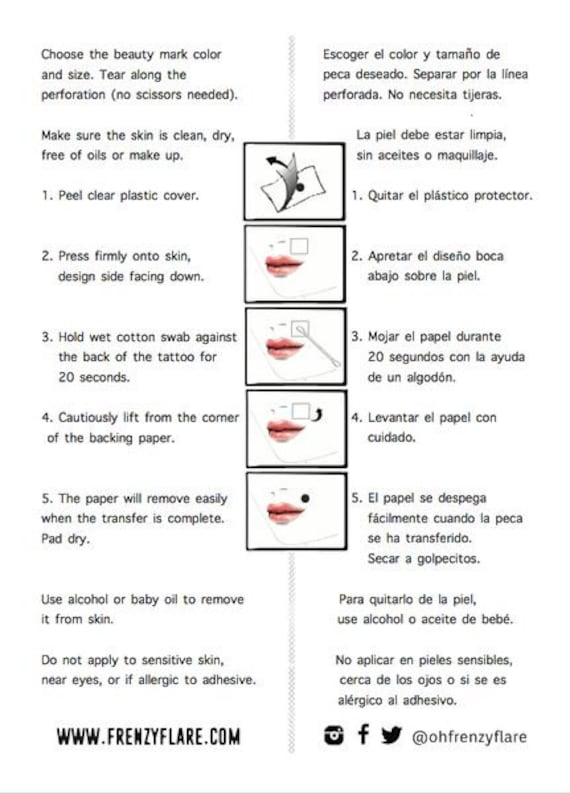This image shows detailed instructions for applying a beauty mark, provided by www.FrenzyFlare.com. The setup on a plain white background features two columns of text—English on the left and Spanish on the right—with step-by-step illustrations in five black-outlined boxes running down the center. At the top left, the instructions begin in small black letters, outlining steps such as selecting the beauty mark color and size, and tearing along the perforation without the need for scissors. The text advises ensuring that the skin is clean, dry, and free from oils or makeup. 

The step-by-step guide follows: 
1. Peel the clear plastic cover.
2. Press the design firmly onto the skin, facing down.
3. Hold a wet cotton swab against the back of the tattoo for 20 seconds.
4. Carefully lift from the corner of the backing paper.
5. The backing paper will remove easily once the transfer is complete; pat dry.

The five illustrations demonstrate these steps with visual aids that include the image of a woman’s nose and lips, and the position of the beauty mark near her mouth. Additional instructions mention using alcohol or baby oil for removal, and warn against applying the product to sensitive skin, near the eyes, or if allergic to adhesive. At the bottom left, the website www.FrenzyFlare.com is printed in black text, and at the bottom right, there are icons for Facebook and Twitter alongside the handle @FrenzyFlare.